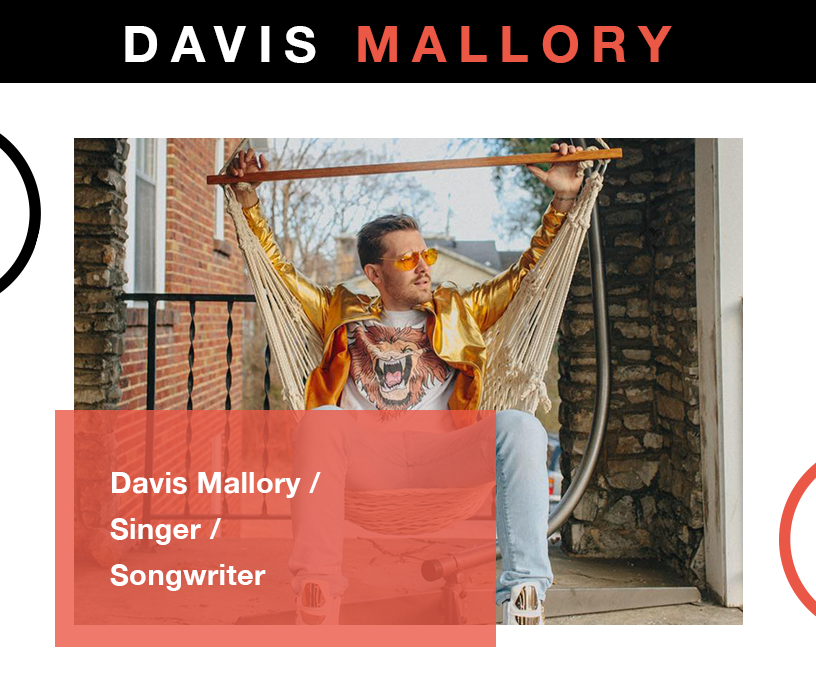The image appears to be a PowerPoint slide featuring Davis Mallory. At the top, "Davis Mallory" is written in all capital letters on a black banner, with "Davis" in white text and "Mallory" in red text. Below this, there's a color photograph of Davis Mallory sitting in a beige rope hammock, which gives the appearance of a chair, likely positioned on a porch or an outdoor balcony. The porch features stone walls and a black wrought iron railing. Davis is styled with his hair slicked back, wearing orange, almost goldish, sunglasses, a flamboyant gold jacket, light-colored jeans, and a t-shirt adorned with a roaring lion's head. In the lower left corner of the image, another text banner appears, consisting of white text on a transparent orange background, which reads: "Davis Mallory / singer / songwriter."